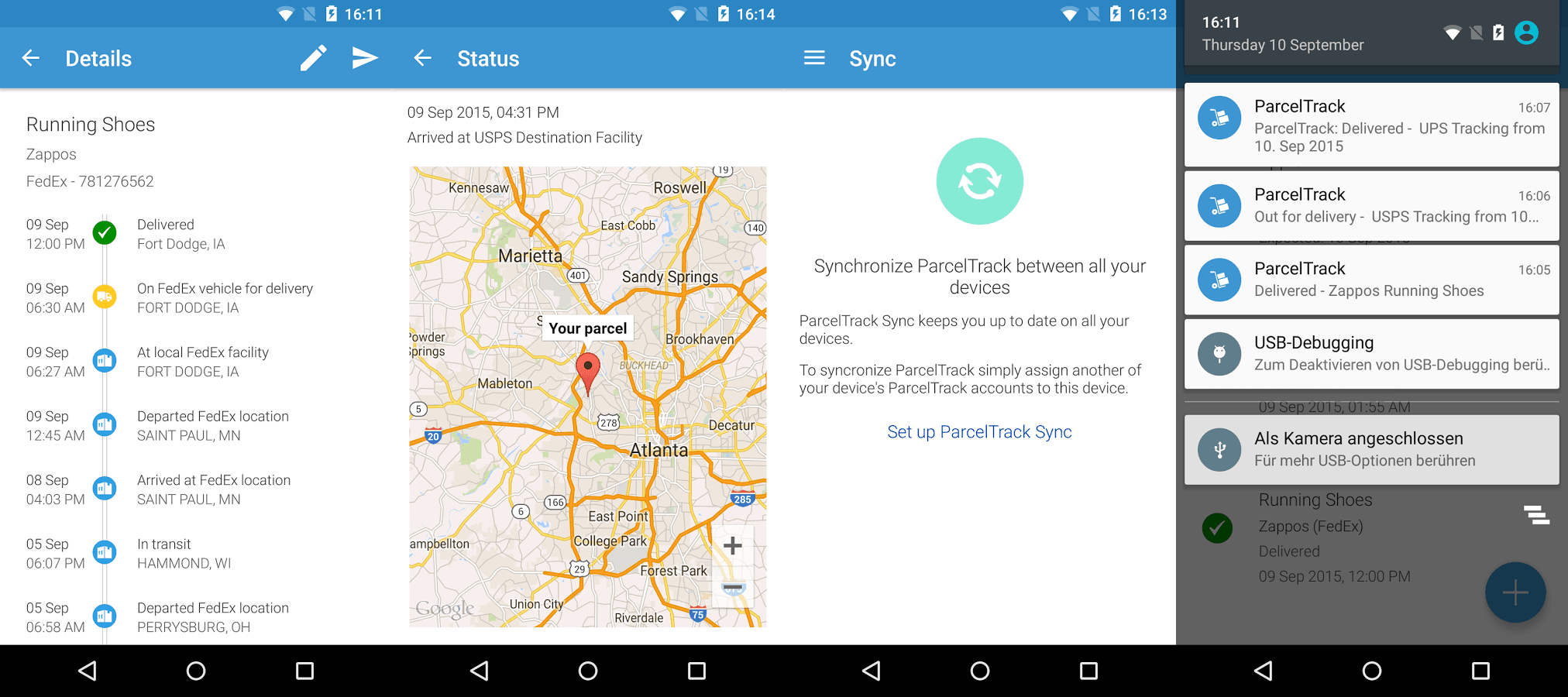**Detailed Caption:**

This smartphone screenshot displays a delivery tracking update for a shipment of running shoes from Zappos, via FedEx. The time on the phone reads 16:11, and below that, a blue section with the label "Details" is shown along with a pencil icon and a forward icon indicating "Status and Sync." On the left, the key details of the package's journey are outlined: 

- The package is listed as "Running Shoes, Zappos, FedEx."
- Updates from the delivery company are specified: 
  - Delivered in Fort Dodge, Iowa.
  - On a FedEx vehicle for delivery at the local FedEx facility in Fort Dodge, Iowa.
  - Departed from the FedEx location in St. Paul, Minnesota.
  - Arrived at the FedEx location in St. Paul, Minnesota.
  - In transit from Hammond, Wisconsin.

On the right side of the screen, there's a map with a red location pin indicating "Your Parcel." Adjacent to this, there is a section urging the user to "Synchronize parcel track between all your devices," followed by a blue hyperlink prompting the user to "Set up parcel track sync." The screenshot is slightly blurry, making some small text hard to read clearly.